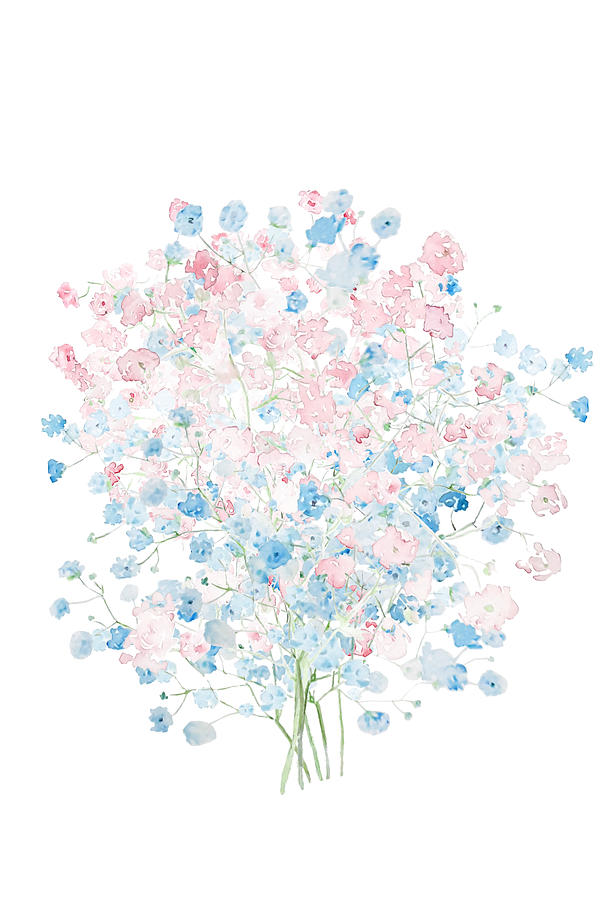The painting is a delicate watercolor depiction of a bouquet of flowers set against a plain white background with no visible borders. At the base of the composition, there are six very thin green stalks, each measuring about a quarter to half an inch in height. These stalks give rise to an intricate network of finer, light green branches that wind their way through the arrangement.

The focal point of the image is a densely packed cluster of small flowers, each about an eighth to a quarter of an inch in size. The flowers, which are a mix of light pink and light blue, are beautifully interspersed and create a frilly, bushel-like appearance. Some blooms are slightly darker pink or blue due to overlapping watercolor layers.

This rounded bouquet occupies the entirety of the painting, with the green branches sporadically visible amidst the predominantly colored scene. The overall impression is a soft, ethereal burst of color, with the delicate nature of the watercolor medium adding to its charm. The image gives a sense of completeness even though it is cut off at the bottom, leaving out any ground or surrounding elements.